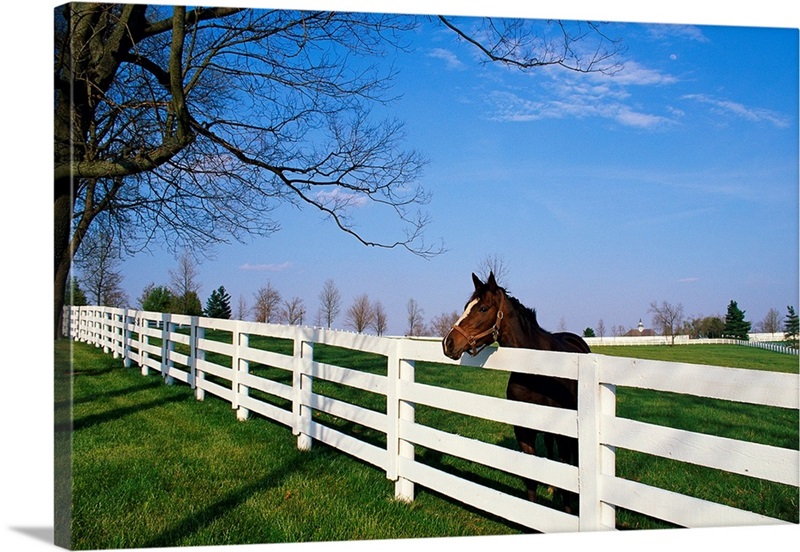In this captivating photograph, a brown horse with a distinctive white blaze on its forehead leans over a white wooden fence. The setting is a beautifully manicured field with vibrant shades of green grass stretching into the distance. Above, a clear blue sky, adorned with traces of white clouds, creates a serene backdrop. Despite the season suggested by the barren tree branches, likely indicating late winter or early spring, the scene feels warm and inviting. The horse appears to be gazing pensively beyond the fence, adding a touch of contemplative grace to the image. In the distant background, a treeline and the faint tip of a church spire are visible, further enhancing the pastoral charm. The detailed white fence extending far back suggests this may be a fancy stable or racetrack, completing the picturesque setting.